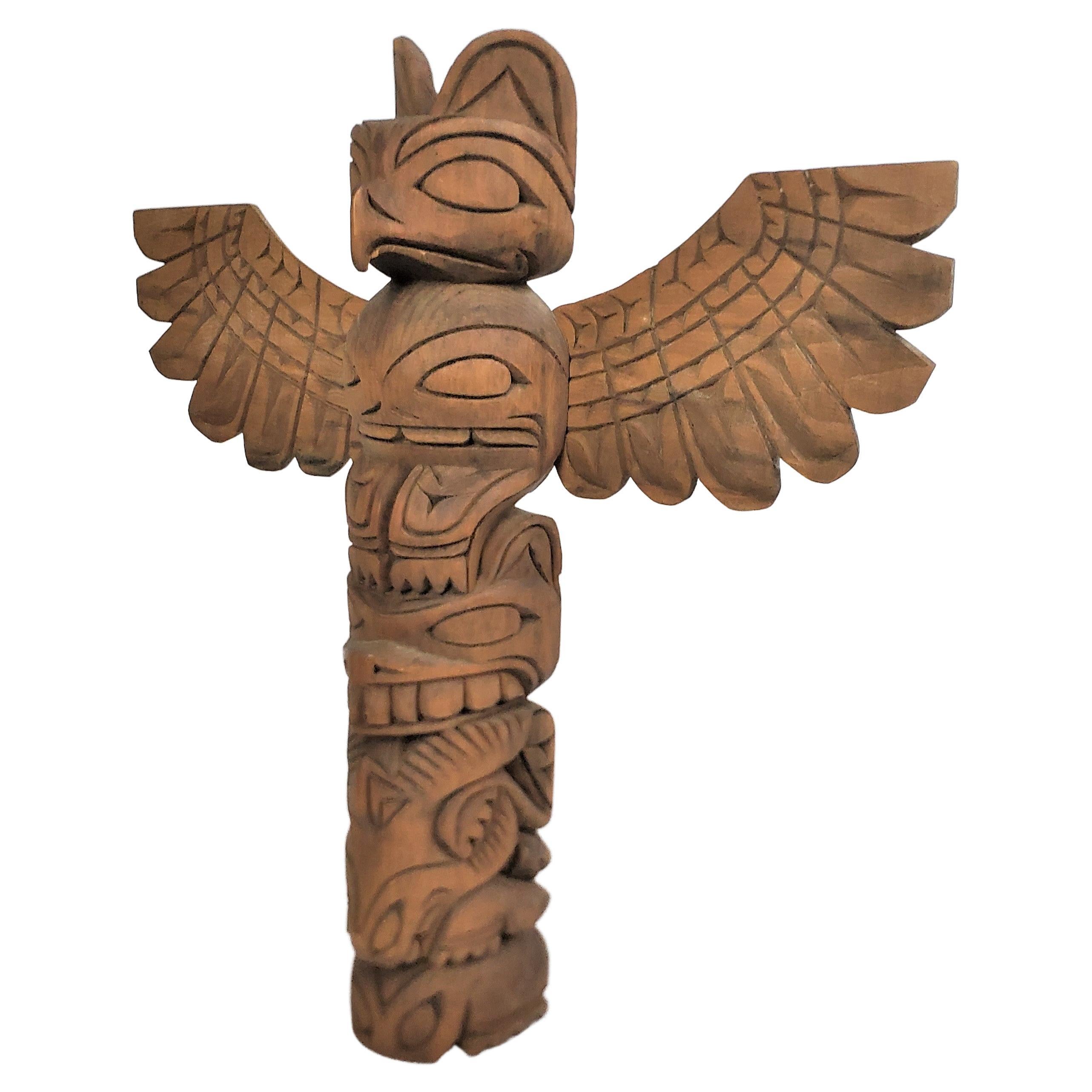The image depicts a carved wooden totem pole set against a plain white background, showcasing intricate Native American designs. The totem pole, medium brown in color and unpainted, features multiple faces and creatures stacked vertically, each representing various animals through distinctive characteristics such as beaks, horns, and teeth. At the top of the totem pole is a face resembling an eagle with prominent ears. Below it, there is a small face with giant teeth and feet, possibly a reference to a turtle with its legs poking out. The following section resembles a dragon, while the next one down features a ram with distinct sheep-like horns. The very bottom face may represent a smaller animal like a rabbit or rodent. Dramatic wings extend outward from the sides of the totem, further enhancing its imposing and fantastical appearance.